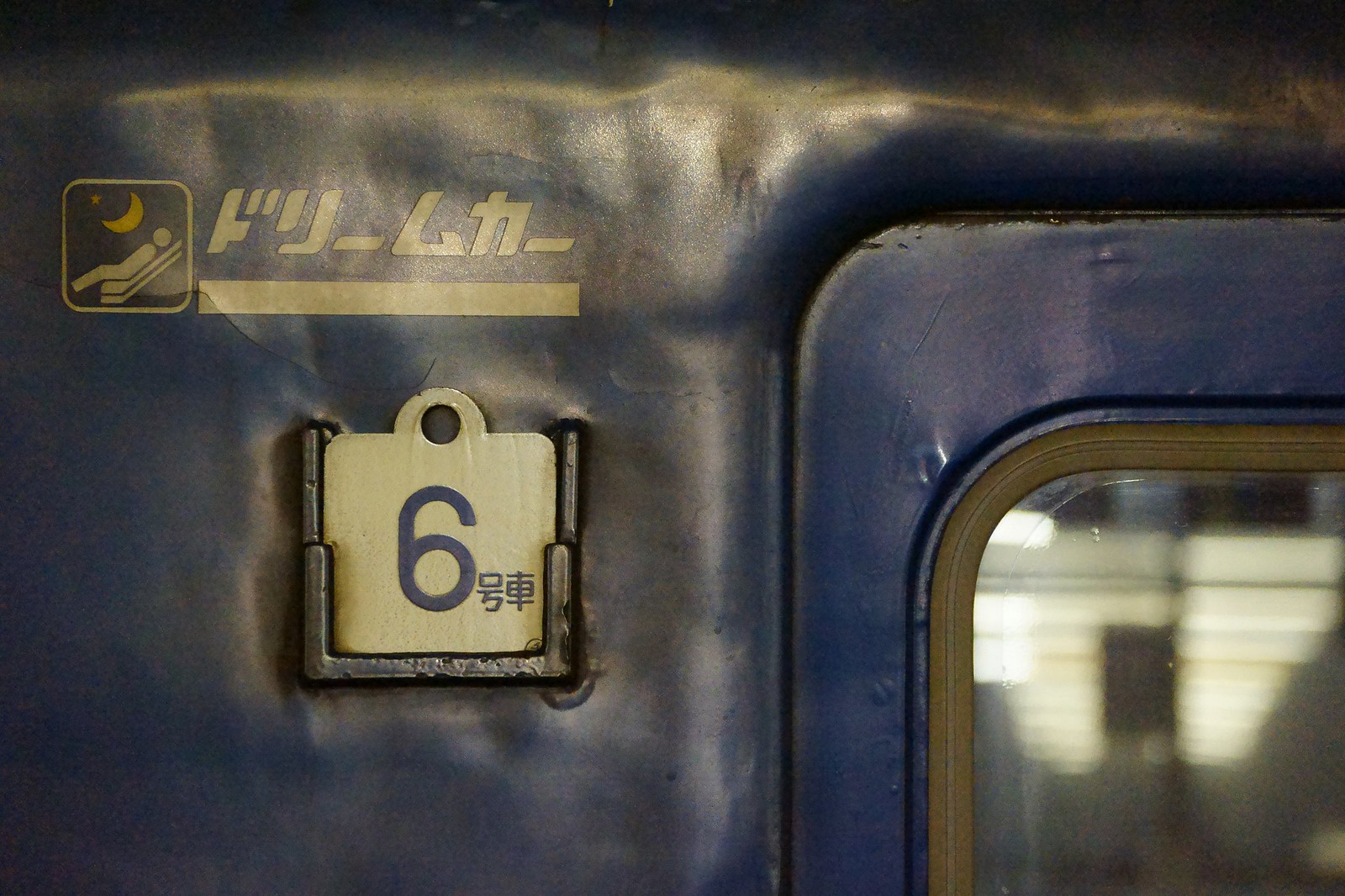This indoor color photograph is a close-up of a battered and dented train's blue exterior. Dominating the frame, the focal point is the side panel of the train. On the left, there is a notable logo featuring a stylized reclining figure with a crescent moon above their head, likely indicating a sleeper car. Accompanying this logo is some foreign writing, possibly in Arabic or an Asian script, which may offer further context or instructions. Positioned directly below the logo, a silver metal plate is prominently affixed, bearing the number six, and additional characters that might be Korean suggesting it's part of a changeable indicator system. On the right side, the upper-left corner of a metallic door is visible, edged in beige and blue. The door includes a small glass pane in the lower right corner, harmonizing with the overall blue hue and contributing to the utilitarian design of the weathered train car.